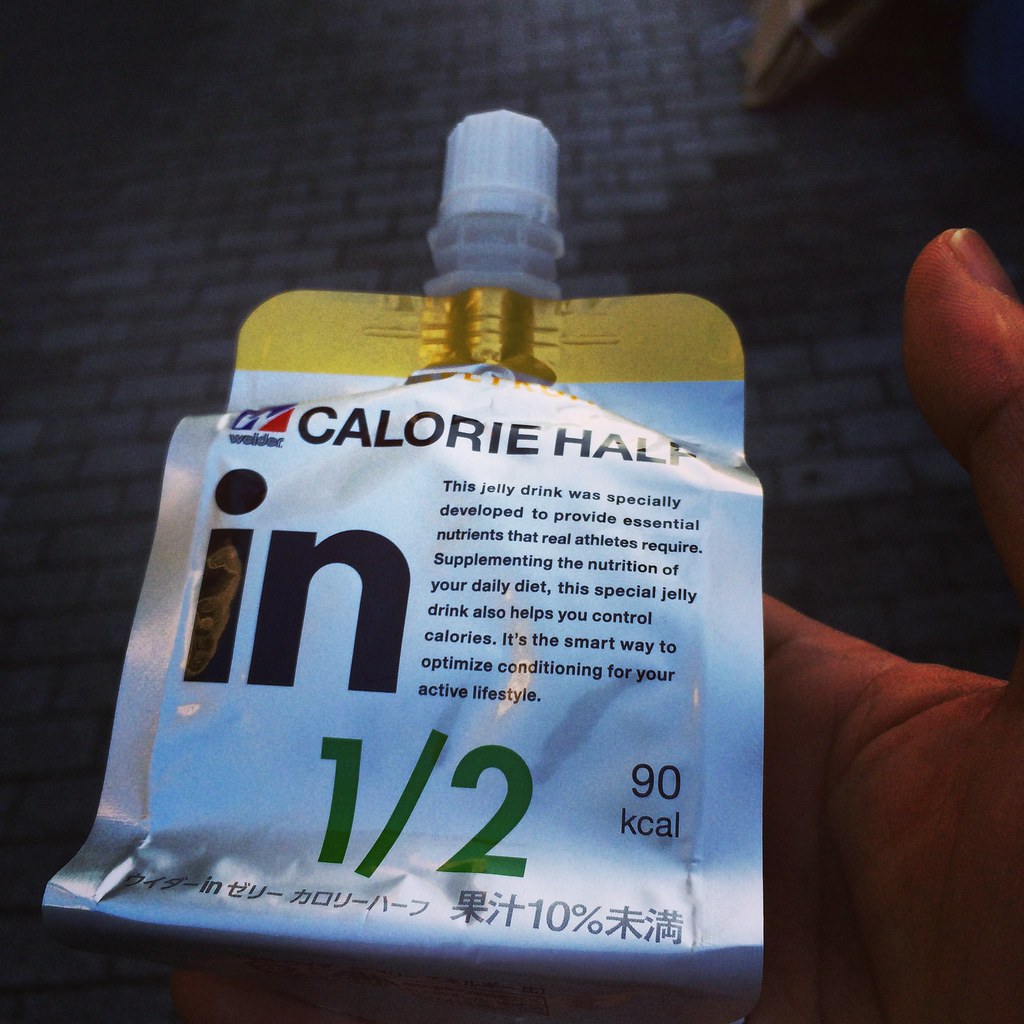The image features a product pouch prominently displayed in the center, adorned with a bright yellow lip at the top and sealed with a plastic cap. The upper part of the pouch is labeled with the text, "Calorie Half," accompanied by an adjacent, indistinct symbol on the left. 

The main body of the pouch carries a detailed description in the middle, stating: "This jelly drink was specially developed to provide essential nutrients that real athletes require. By supplementing the nutrition of a daily diet, this special jelly drink also helps you control calories. It's a smart way to optimize conditioning for your active lifestyle."

On the left side of the pouch, large, bold black text highlights the words "One Half." Directly to the right, the pouch indicates that the contents provide "90 kilocalories." Additionally, there are some Asian characters—possibly Japanese or Chinese—printed on the pouch in silver ink, lining both the left and right sides. The backdrop of the image appears to be a rustic brick floor, providing a contrasting texture to the sleek, modern look of the jelly drink pouch.